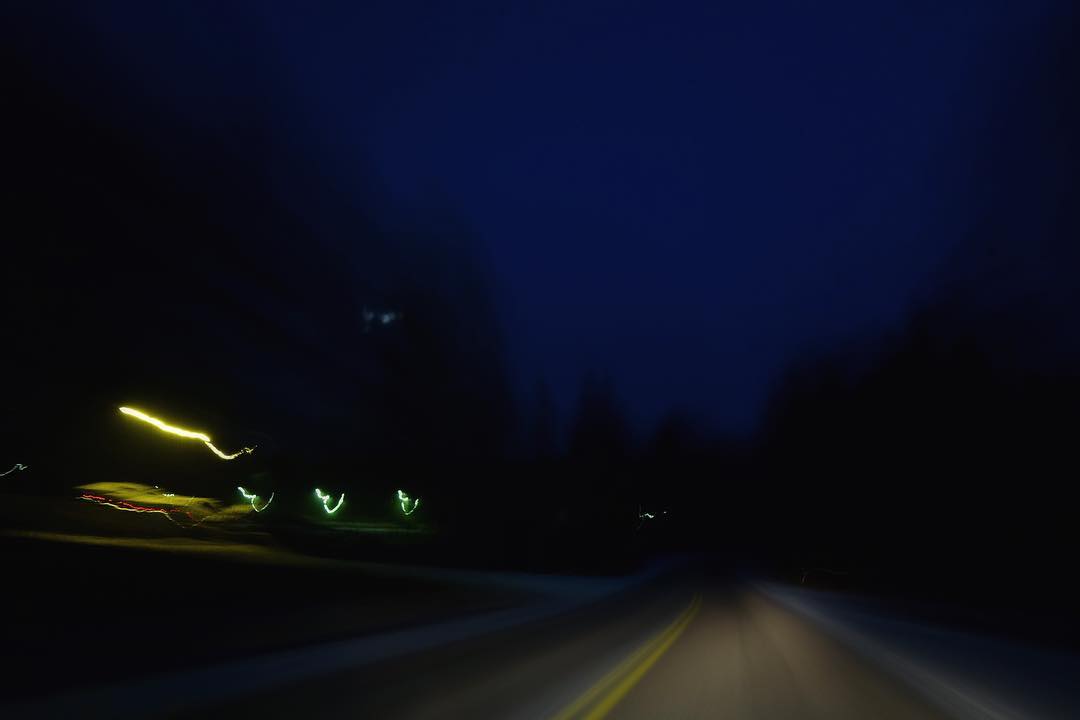Captured through a windshield at nighttime, this image showcases a dimly lit two-lane highway. The road is marked by prominent double yellow lines in the middle and bears the faint traces of tire marks on its asphalt surface. The scene is enveloped in a pitch-dark night sky devoid of stars or clouds, creating an almost eerie atmosphere. Silhouettes of tall pine trees stand sentinel on either side of the road, their outlines dark and foreboding. To the left, reflections of distant lights manifest as elongated streaks and cupped shapes that are distinctly yellow and white, though blurred and unfocused. The image is primarily illuminated by the car's headlights, casting a stark beam of light that highlights the path ahead amidst the enveloping darkness.